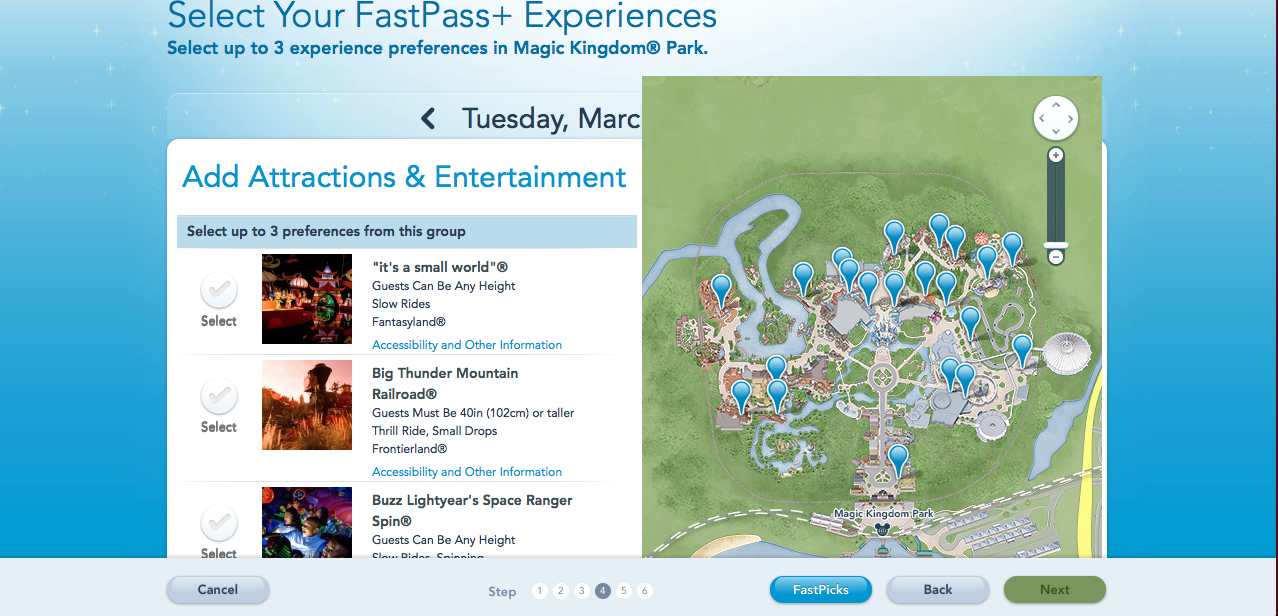The image captures a detailed screenshot of the Disney Magic Kingdom's FastPass+ selection screen. The interface prompts the user to "Select Your FastPass+ Experience" at the top, allowing them to choose up to three experiences within the Magic Kingdom Park™. Although the exact date is partially obscured by a park map with blue markers indicating various attractions, what is visible indicates it is a Tuesday in March.

On the right side of the screen, the park map features clickable blue tabs scattered across various sections. The left side showcases three available rides for selection: "It's a Small World," "Big Thunder Mountain Railroad," and "Buzz Lightyear's Space Ranger Spin." Additionally, there is a checkbox feature on the right side next to a button, allowing users to confirm their selections.

At the bottom of the screen, a progress indicator reveals that the user is on one of five steps in the process of securing their FastPass+ reservations. This comprehensive layout conveys both the interactive and informative elements of planning a visit to the Magic Kingdom.